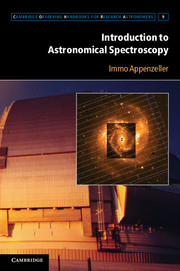The image, resembling a small thumbnail of a textbook cover, prominently features the title "Introduction to Astronomical Spectroscopy" in white font at the top. Directly underneath, the author's name, "Immo Appenzeller," is displayed in golden writing. The cover design includes a black banner at the bottom left corner with indistinct white text, likely starting with the letter "C," possibly indicating "Cambridge University Press."

The visual elements consist of two overlapping images. The primary image depicts an industrial-looking structure, possibly an observatory, in rich shades of purple, gold, and reddish tones. A secondary, smaller inset image showcases a cosmic scene with dazzling, golden, glittery lights, resembling either a star formation or an asteroid, emitting bright, fiery colors in a spiral pattern. The overall background and some structural elements convey a dark purplish-blue hue, contributing to the celestial theme of the cover.